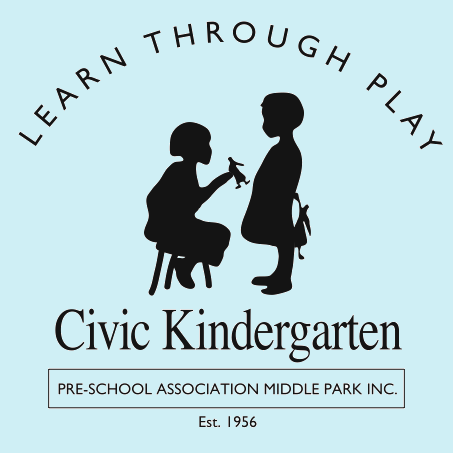The square poster features a light baby blue background. At the top, the title "Learn Through Play" is elegantly arched from left to right in black ink, reaching its peak in the center of the poster before descending symmetrically. Beneath the title, there are two black silhouette figures of children. The child on the left, assumed to be a girl wearing a dress, is seated on a stool and holding a doll. Opposite her stands another child, also in a dress, holding the same doll behind her. Below this scene, the text reads "Civic Kindergarten" in black letters. Encased in a black-outlined rectangle further below, it says "Preschool Association, Middle Park, Inc. Established 1956." The image strongly evokes a sense of learning and play, likely an advertisement or informational pamphlet for the organization.